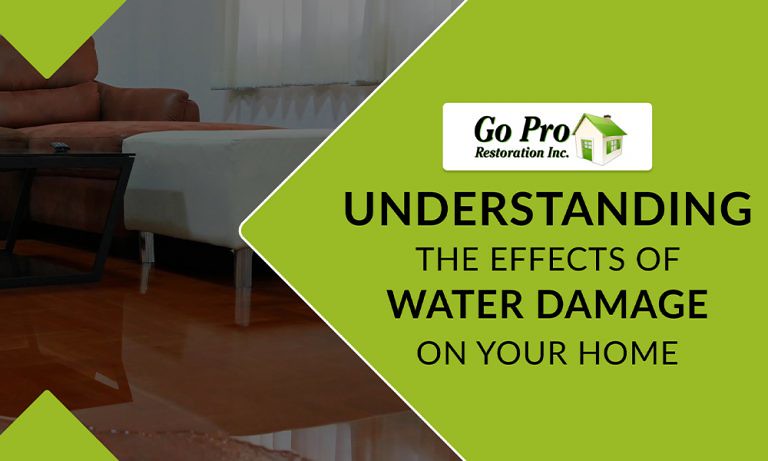This image appears to be a slide from a promotional presentation by GoPro Restoration Inc. On the left side, a photograph shows a living room with shiny wooden floors, partially covered in water, indicating water damage. A couch is visible in the backdrop, with an X shape overlaying the photograph and a dark semi-transparent shade adding emphasis. The right side features a green backdrop with a thin white border, displaying the GoPro Restoration Inc. logo at the top alongside a small house icon. Below the logo, in large black text, it reads, "Understanding the effects of water damage on your home," providing information on water damage restoration.